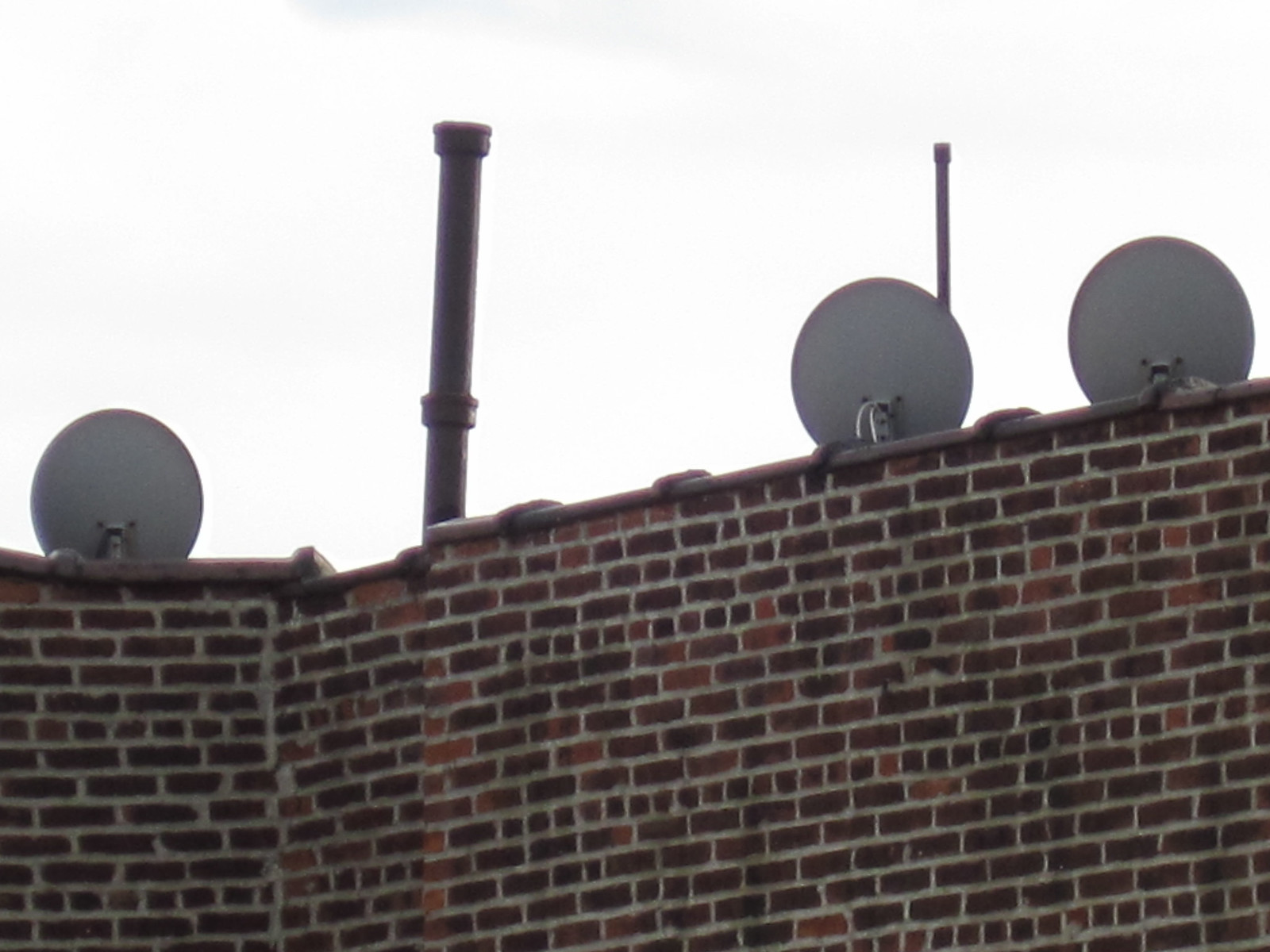In the photograph, a brick wall is seen with dark brown and deep orange bricks, interspersed with a few lighter shades. The bricks are held together by a gray or off-white caulking. Along the top edge of the wall is a brown rim or rod. Attached to and above the wall are three gray satellite dishes, two clustered towards the right and one towards the left. At the top center of the wall, a large black pole extends upwards. The backdrop behind the satellites and the pole is a bright, completely white sky, giving the impression of a very sunny day with no visible blue in the sky.